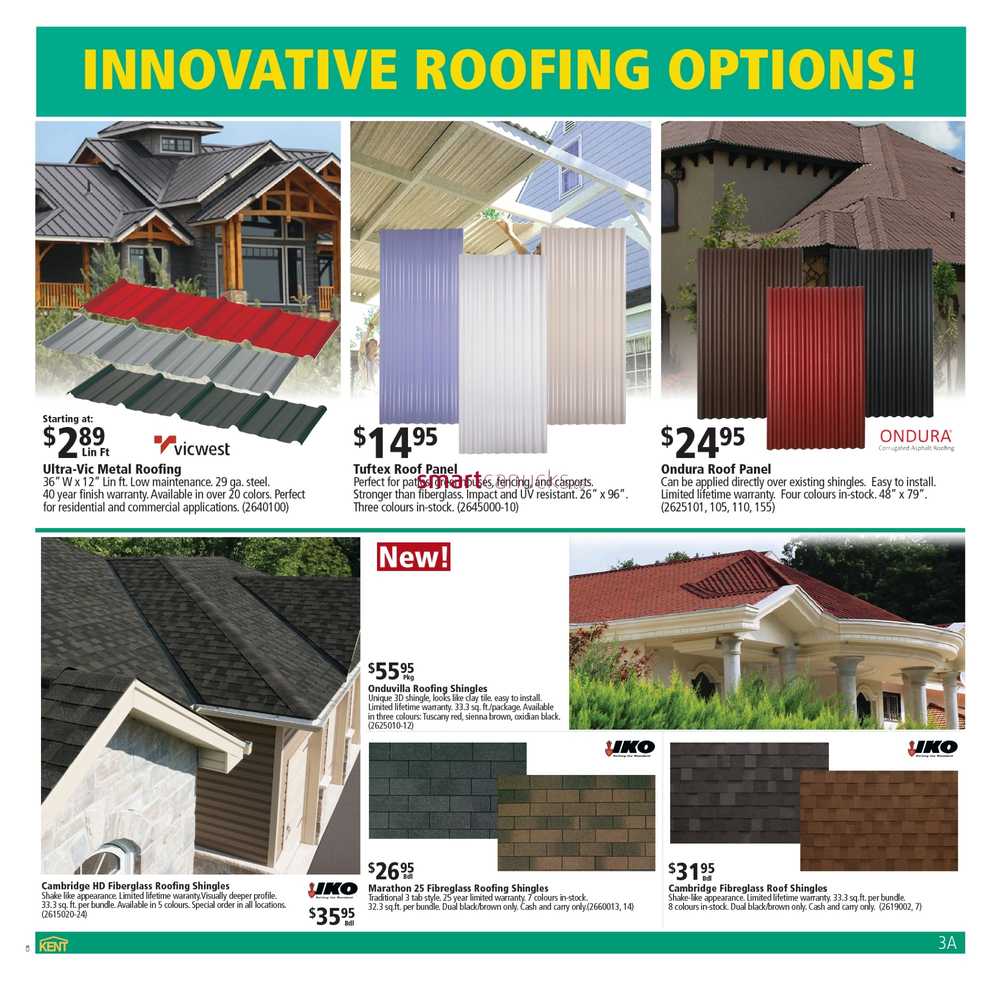**Detailed Caption:**

This image is a screenshot of a hardware shop advertisement page, showcasing various roofing options. At the very top, there's a prominent green bar with bold, yellow uppercase letters reading "INNOVATIVE ROOFING OPTIONS!" Below this banner, the page is divided into five distinct advertisement sections.

**Top Half (Three Rectangular Boxes):**

1. **Top Left Box:**
   - **Image:** A modern cabin-like house with a roof featuring multiple angles and heights.
   - **Ad Details:** 
     - **Price:** Starting at $2.89 per linear foot.
     - **Brand:** Vicwest (spelled "Vic West")
     - **Product Description:** UltraVic Metal Roofing, dimensions 36 inches wide by 12 feet in linear length, made of low maintenance 29 gauge steel with a 40-year finish warranty. Available in 20 colors. Further small text includes "low maintenance 29…" but some details are illegible.

2. **Top Center Box:**
   - **Image:** The top of a white carport, showing the underside of its roof panels.
   - **Ad Details:**
     - **Price:** $14.95 per unit.
     - **Product:** Tuftex Roof Panels.
     - **Additional Information:** Described as stronger than fiberglass and UV resistant, with dimensions of 26 inches by 96 inches. A red marker labeled "Smart" partially obscures some text.

3. **Top Right Box:**
   - **Ad Details:**
     - **Price:** $24.95 per unit.
     - **Brand:** Ondura 
     - **Product:** Ondura Roof Panels.
     - **Image:** A roof with brown panels on a tan stucco-finished house.
     - **Additional Information:** The panels can be applied directly over existing shingles, are easy to install, and come with a limited lifetime warranty.

**Bottom Half:**

4. **Bottom Left Box:**
   - **Image:** A gray-shingled roof with varying heights.
   - **Ad Details:**
     - **Product:** Cambridge HD Fiberglass Roofing Shingles.
     - **Price:** $35.95 per bundle (or roll, text is slightly unclear).

5. **Bottom Right Box:**
   - **Image:** A building with white pillars and a bright red roof.
   - **Ad Details:**
     - **Product:** Onduvilla Roofing Shingles at $55.95 per package.
     - **Additional Products:**
       - **Marathon Roofing Shingles:** $26.95 per package.
       - **Cambridge Fiberglass Roofing Shingles:** $31.95 per package.

This detailed breakdown highlights the variety of roofing products available, their costs, and specific features, providing potential customers with comprehensive choices for their roofing needs.